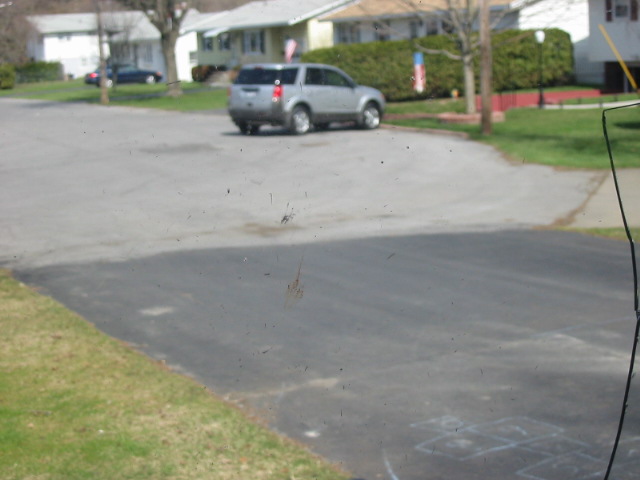The image depicts a dark gray driveway situated in a cul-de-sac. Although the photo is of low quality and entirely out of focus, various elements are discernible. There is no vehicle parked on the driveway, which is flanked by patches of grass on both the left and right sides. In the bottom right corner, blue chalk markings outline a hopscotch pattern on the driveway. A car is either pulling out of a nearby driveway or exiting down the road, visible in the background. Additionally, several houses line the street, contributing to the residential ambiance of the scene.